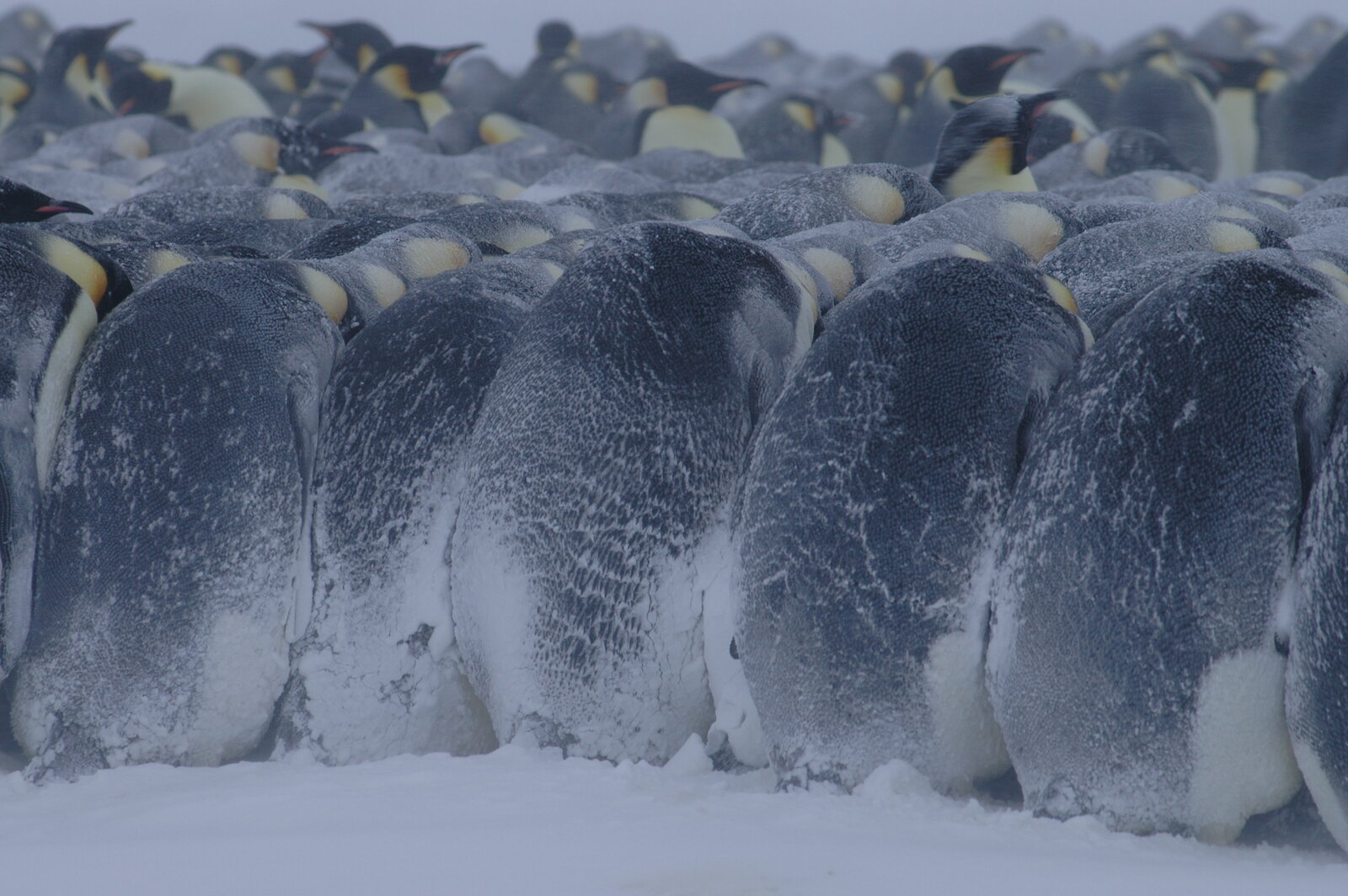In this captivating outdoor photograph, a mass of penguins huddle together on the snow-covered ground, likely taken by a professional wildlife photographer. The penguins, numbering in the dozens, present a striking scene of black-and-white figures against the stark white backdrop of their natural habitat. With their bodies clustered tightly, some of the penguins in the foreground have their heads ducked, as if bracing against the cold or seeking comfort from one another. Others in the background have their beaks raised, revealing black-topped heads and distinctive golden-yellow accents beneath their chins, which contrast with their otherwise monochromatic coloring. The image, devoid of any other animals or text, offers a glimpse into the penguins' social behavior, possibly for warmth or social interaction, engrossing viewers in the life of these fascinating creatures in their snowy world.